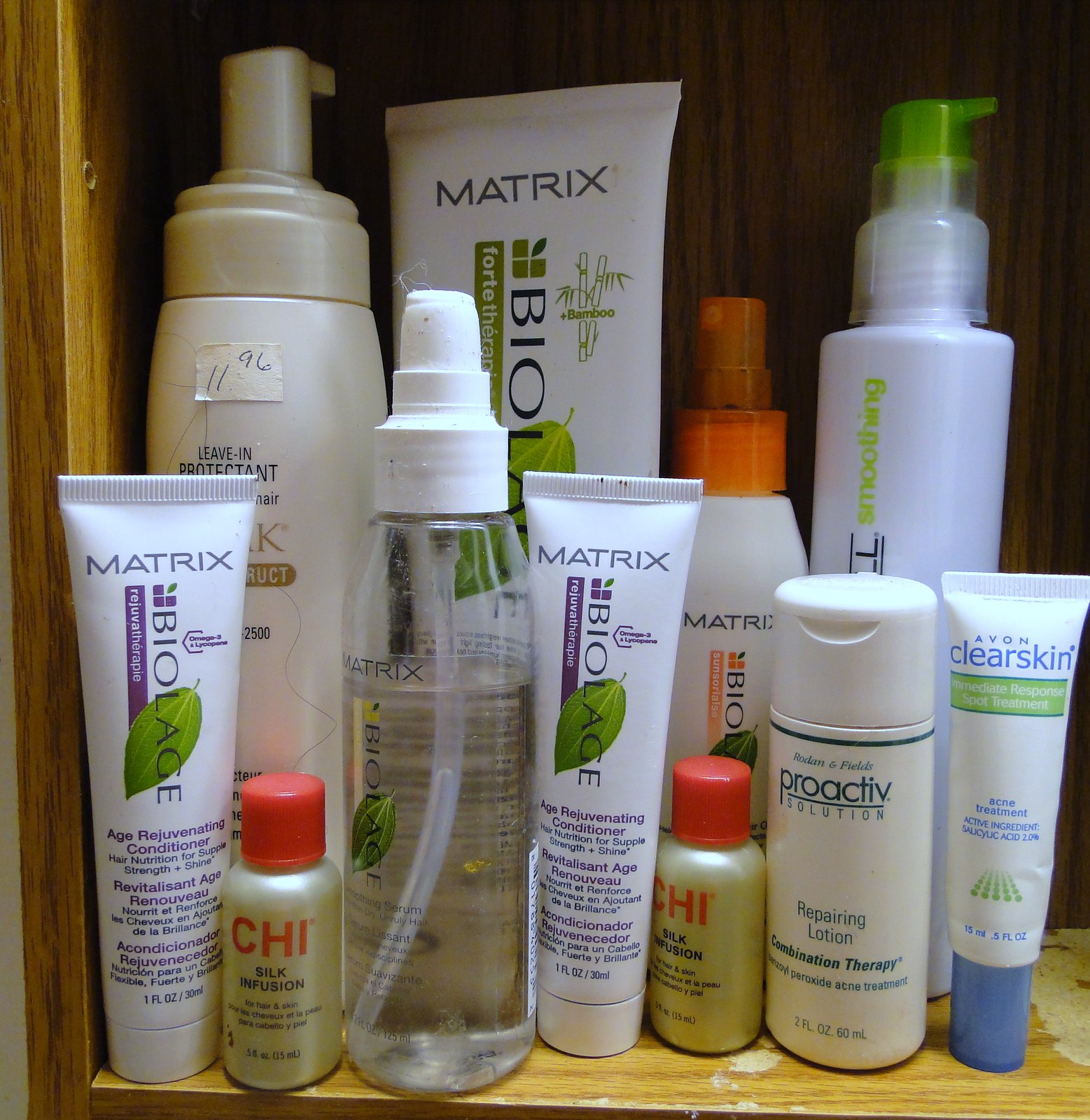The photo captures a well-stocked personal care cabinet, filled predominantly with white containers of various products. In the foreground, there are two tubes of Matrix Biolage Rejuvena Therapy, an Age Rejuvenating Conditioner that promises to provide hair nutrition for supple strength and shine. The product description is also written in Spanish. Another tube from the Matrix Biolage line is partially visible in the background, with legible text indicating it derives benefits from bamboo and mentions something related to strength in Spanish.

On the bottom right sits a tube of Avon Clear Skin Acne Treatment upright. To its left, there is a smaller tube labeled Proactiv Solution Repairing Lotion, part of a Combination Therapy line. Several other Matrix products are also present, including two smaller bottles of what appears to be Margie Silk Infusion, though their labels are mostly obscured. Additionally, a clear plastic bottle with the Matrix Biolage label is visible, but its specific product name is not discernible. In the back of the cabinet, there's a bottle labeled Leave-In Protectant, which seems to be a hair product as well.